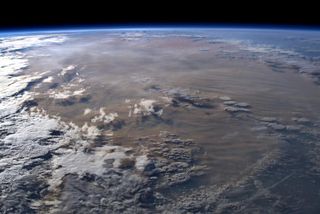A stunning, high-resolution image captures a close-up view of Earth from outer space, likely taken from a space station. It showcases a segment of the Earth's surface with distinct terrain elements. The curvature of the planet is highlighted by a glowing, light blue halo at the horizon, contrasting sharply with the blackness of space in the backdrop. The image features a mix of colors: varying browns and greens convey the land, while blue tones represent the surrounding ocean. White and gray clouds are scattered predominantly to the left side, appearing curly and dynamic against the earth's surface. The absence of text, people, and man-made structures emphasizes the natural beauty of our planet. The sunlight enhancing the left side of the image further adds depth and dimension to this captivating view from space.